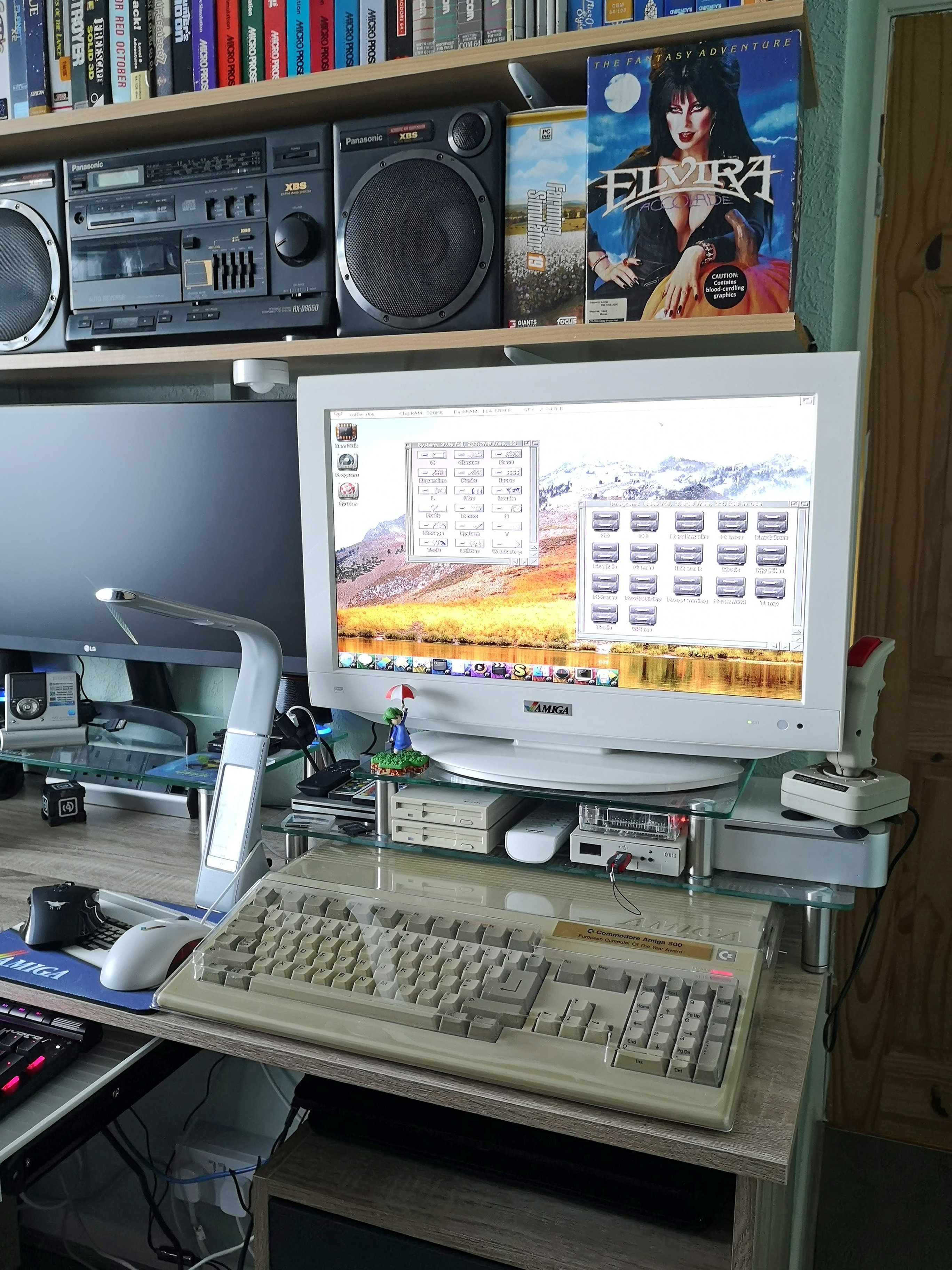The photograph showcases a detailed view of a vintage home office workstation. The central focus is an old desktop computer setup complete with a white monitor and a gray, 80s-style keyboard. There are multiple disk drives and hard drives on the desk, along with a blue mouse pad, two mice, and a video game controller. The background features a screensaver depicting a mountain range with orange hues at the bottom and white-capped peaks.

Above the monitor, an elaborate shelving unit painted rich forest green holds various items, including a distinct black boom box with a tape and CD player flanked by two black speakers. Prominently displayed on the middle shelf is a partially visible DVD cover of Elvira. Surrounding the boom box is an arrangement of books stretching from the upper right to the upper center of the shelf. The shelf is made of wood.

To the left of the computer, a lamp sits next to the mouse and another black device with red buttons. Additionally, a niche bestseller novel titled "Allura," featuring an illustration of a busty woman with dark brown hair admiring herself in a mirror, is seen on the shelf. You can also discern some faint fluorescent lighting emanating from the top left corner of the image, adding a soft glow to the scene. The entire setup is nestled against a gray wall, underlining the vintage and eclectic ambiance of this home office space.